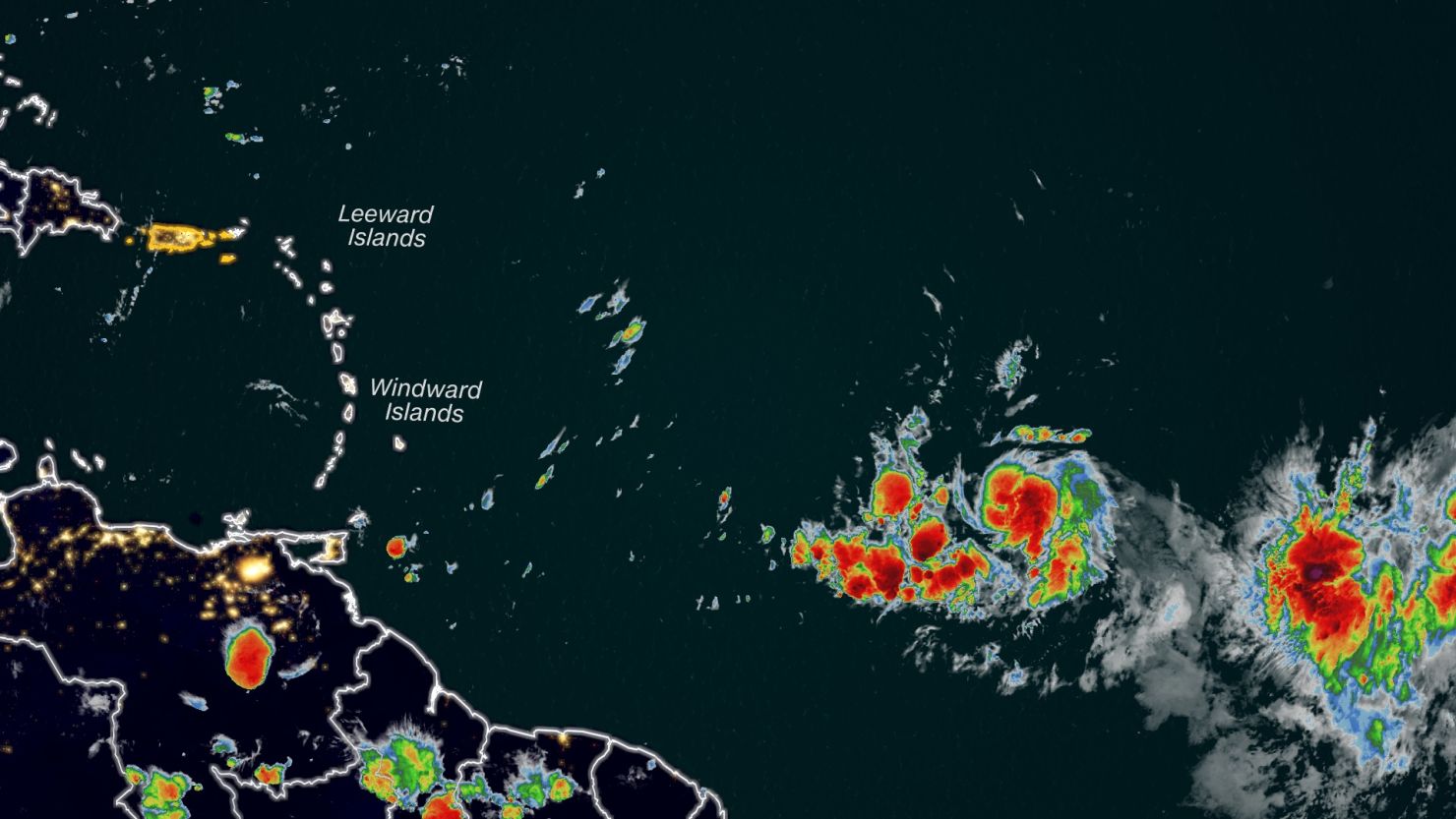The image depicts a highly detailed satellite weather map focusing on a region in the Atlantic Ocean just off the coast of Cuba and the northern part of South America, including notable Caribbean islands such as Puerto Rico and Haiti. The map shows the various land masses and oceanic expanses in black and white, with country borders highlighted in white for clarity. Superimposed on this base are vividly colored weather patterns that illustrate areas of meteorological activity. Intense weather systems are indicated by dark red cores surrounded by brighter red areas, which transition to yellow and green as the intensity diminishes. The map reveals two significant tropical depressions or storms occupying the bottom right-hand corner, suggesting potential hurricane development, and these weather systems are markedly prominent, taking up about a third of the image. Additional storm cells appear scattered over the land masses, contributing to the overall concern. Notably, the map labels the leeward and windward islands in the left portion, and despite the absence of numerical data or human figures, the image is crisp and brightly illuminated, likely captured at night due to the visible city lights.